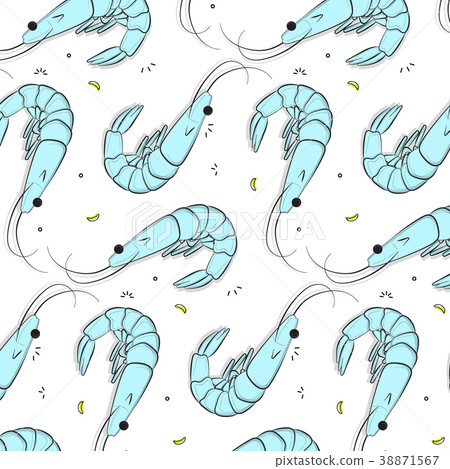This image is a stock illustration featuring multiple cartoon-like blue shrimp arranged in a scattered, repeating pattern against a white background. Each shrimp, colored in a light blue tone and outlined in black, has a segmented body with about five or six sections, resembling rounded, candy-cane shapes. They possess single black dot eyes and two long, black antennae extending from the sides of their mouths. Additionally, the shrimp have small, stem-like appendages for arms. Surrounding the shrimp are small crescent-shaped yellow accents and tiny black lines, adding intricate details to the background. The backdrop also showcases faint gray grid lines crossing it. At the center of the image is a faint watermark reading "Pixta" along with its logo, and at the bottom right corner, there’s text that reads "PixtaStock.com-38871567," giving credit to the source.